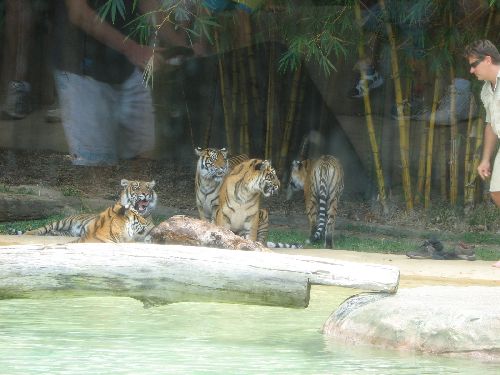The image captures a scene likely set in a zoo, showcasing a group of five tigers in a habitat designed to resemble their natural environment. The tigers, with their striking orange and black-striped coats and white bellies, are positioned in different postures - two are lying down facing each other, while three others are standing, with one turning away from the group. They are surrounded by a pond of green water, where one of the logs is leaning on a grayish stone, and additional logs lay scattered nearby. In the backdrop, there are bamboo trees with leaves cascading down, complementing the more sparsely-packed thinner trees. To the right of the tigers, a man presumed to be a zookeeper stands, identifiable by his sunglasses, white short-sleeved top, and khaki shorts. The setting seems to be viewed through glass, as reflections of people can be seen, reinforcing the zoo-like environment.